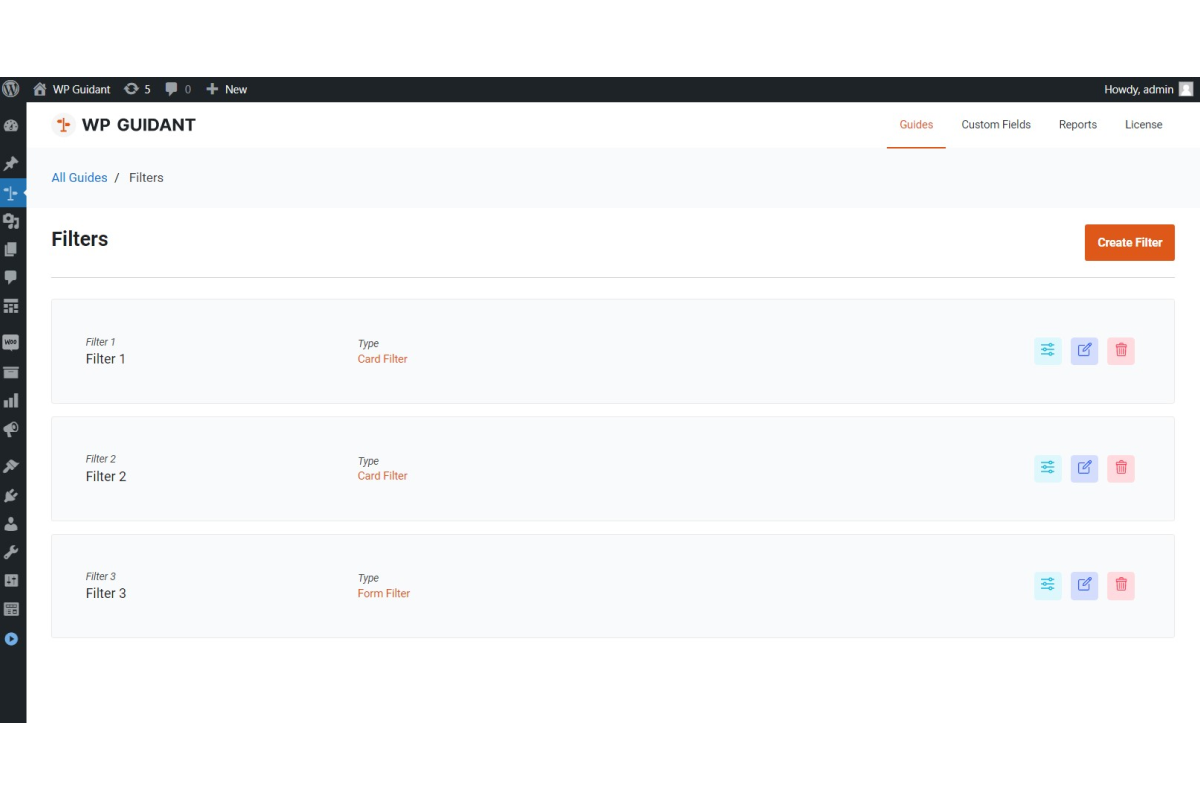The image is a screenshot from a computer or smartphone device, displaying a web interface with a black border at the top and left side. The right and bottom edges blend into the white background of the computer screen. 

On the far left, a vertical black strip hosts multiple icons. At the top, there are several interface elements including an icon labeled "WP Guidant," a chat button, a plus sign with the word "new," and a greeting text "Howdy Admin" next to a gray box containing a white person icon.

The main content area, set against a white background, features various gray boxes and labels. At the upper left corner, "WP Guidant" is prominently displayed. The top-right corner has the word "Guides" highlighted in orange. Below in black text, there are tabs for "Custom Fields," "Reports," and "License." Directly underneath "WP Guidant," the words "All Guides" are shown in blue and "Filters" in bold black. Adjacent to this, a button labeled "Create Filter" is clickable in orange.

The central part of the interface lists three labeled sections: "Filter 1," "Filter 2," and "Filter 3," each described with the terms "Card Filter," "Card Filter," and "Form Filter," respectively. To the right of these sections, three clickable icons are aligned vertically: one green, one blue, and a red trash can icon.